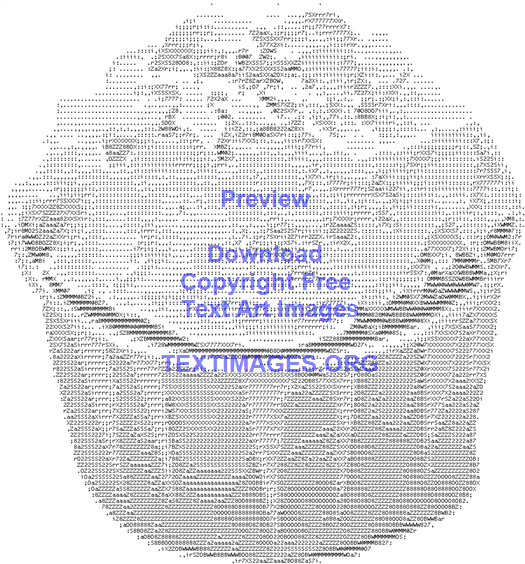This image features a meticulously crafted digital art piece, depicting a cupcake formed entirely by arranging numbers in a structured pattern. The numbers create a detailed grayscale representation, resulting in a grey and white cupcake against a pristine white background. This art piece employs a pixelated style, reminiscent of ASCII art. Superimposed on this number-based cupcake are several lines of text written in blue, reading: "Preview," "Download," "Copyright Free," "Text Art Images," and "textimages.org." The text is neatly organized in rows, and despite its computerized creation, the cupcake's shape is distinctly recognizable with its rounded base and a heap of frosting on top.